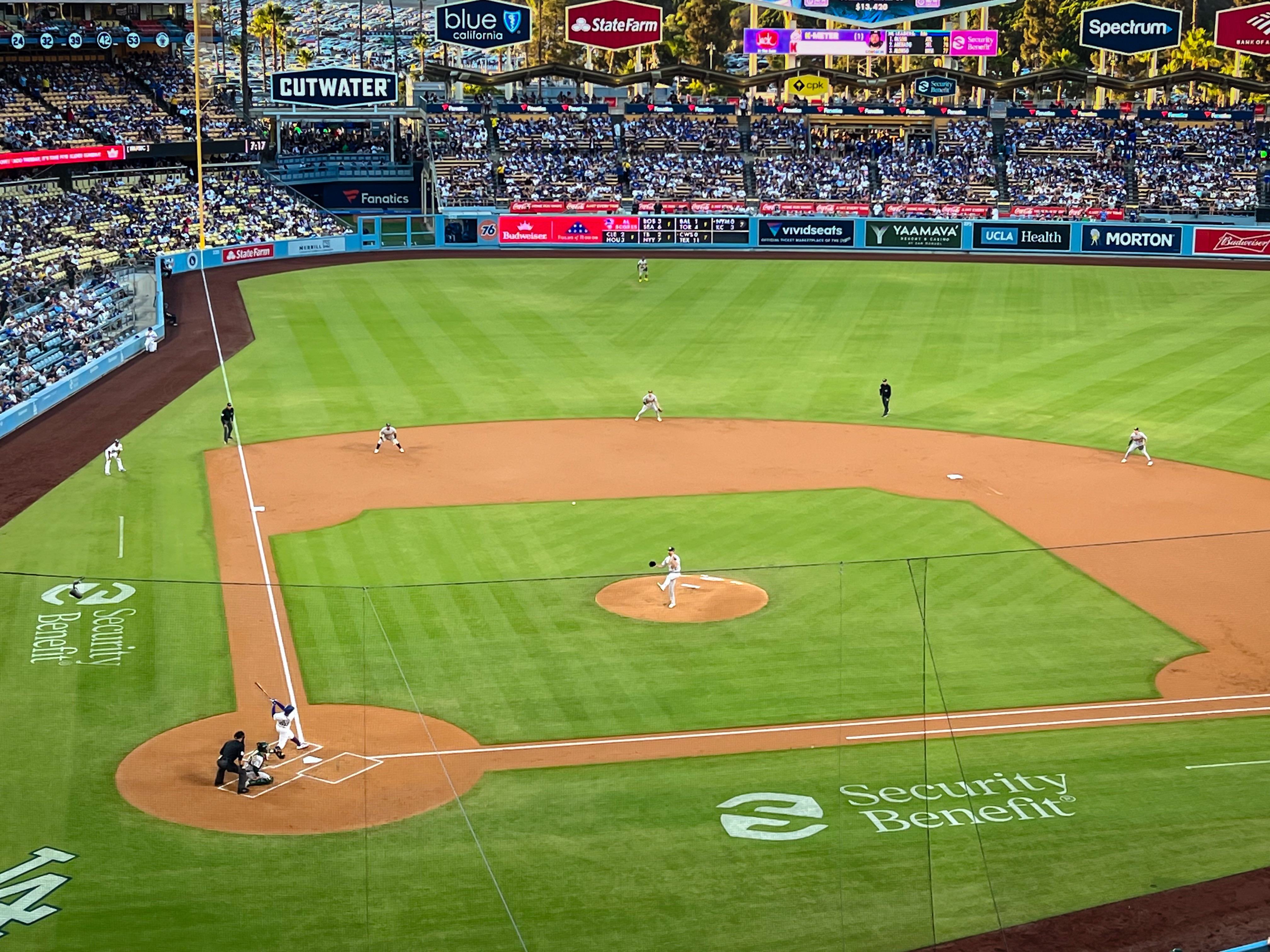The photograph captures a vivid scene from a live Major League Baseball game at Dodger Stadium, viewed from a high vantage point along the first base area. The meticulously maintained green field is highlighted by a light brown, sandy diamond shape and a central pitcher's mound surrounded by green turf. The batter appears to have just swung at the ball, and players are positioned throughout the field. Prominent white text emblazoned on the grass along the edges of the field reads "Security Benefit," signifying a sponsorship. The logo of Security Benefit features a white marking with the letter "S" formed from the green grass. Surrounding the field are multiple tiers of audience seating with foldable yellow and blue seats packed with fans. In the distance, outfield walls are adorned with numerous advertisements from sponsors such as Cutwater, Blue California, State Farm, Spectrum, and Bank of America, adding to the vibrant atmosphere of the stadium.